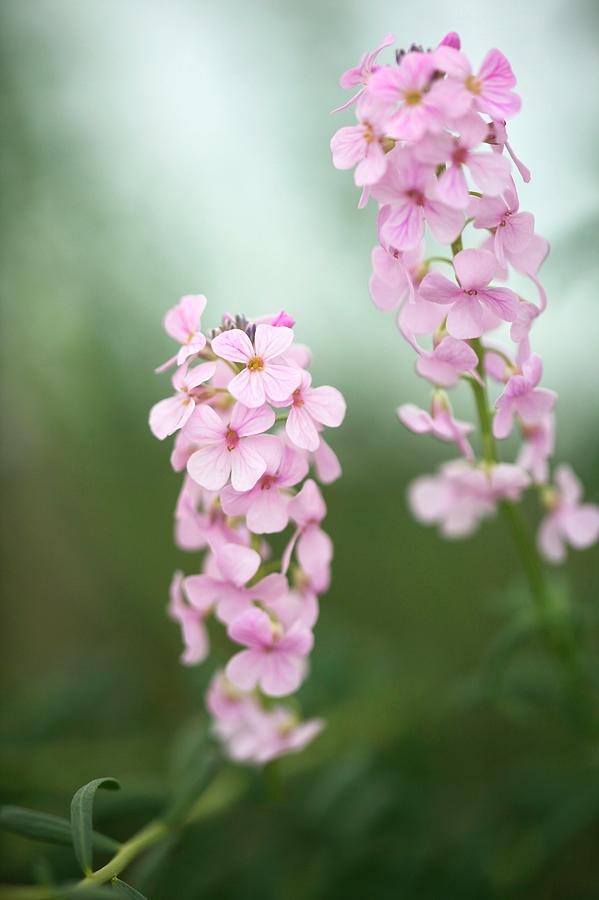This image captures a detailed close-up of two aethionema blooms against a blurred green background, evoking a sense of daytime light. The primary focus is on these two vertically aligned stems:
- The first stem, slightly off-center to the left, extends downwards with its leaves and buds trailing towards the bottom left.
- The second stem starts from the middle right, with budding evident halfway up, reaching towards the top right corner.

Each bloom is composed of clusters of delicate pink flowers, some with touches of pale pink and yellow. The individual flowers within the blooms, possibly peonies, feature small, red dot centers. The thin stems and leaves of the blooms contribute to the overall delicate appearance, with a mix of light and dark green leaves. Despite the blurred background, the clear, focused blooms stand out prominently, making the natural beauty of these flowers the central highlight of the photograph.